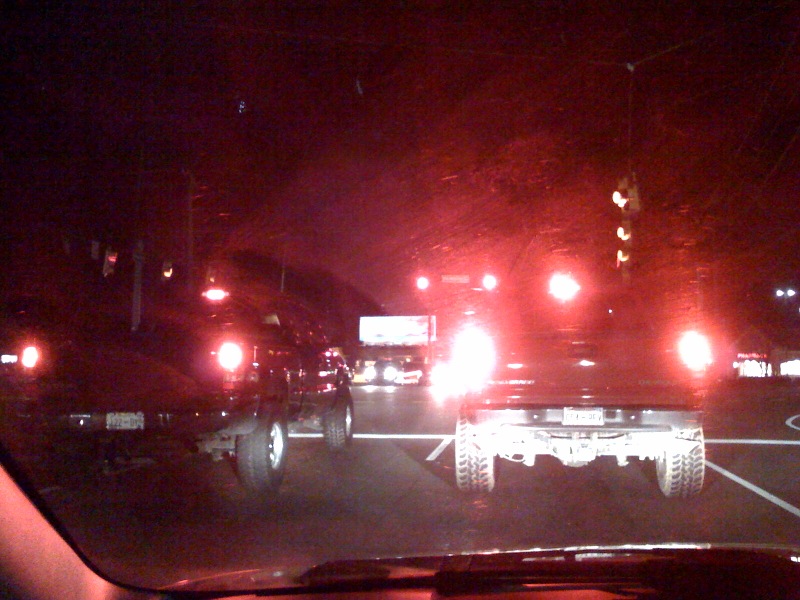A nighttime scene captures the view from a driver's seat, encompassing the lower part of the dashboard and the vehicle's interior frame along the bottom left corner. The road ahead is dimly visible, bathed in the darkness typical of night. Two pickup trucks, one in the same lane and another in the left lane, are halted at a red light, their taillights glowing red and white. Above them hangs a traffic light showing red. Road markings delineate the lanes, and distant headlights signal oncoming traffic. Additional traffic lights in the background cast a faint glow, contrasting with the predominantly black night sky, creating a moody cityscape punctuated by vibrant red lights.